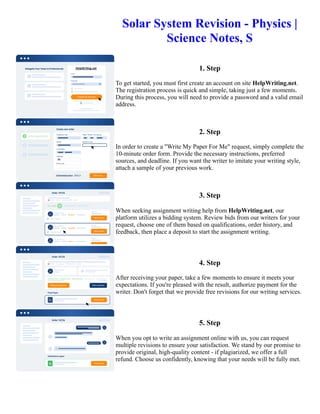The image is a detailed, multi-colored rectangular print piece, likely a pamphlet or a slide focused on Solar System Revision for Physics Science Notes. It consists of two main sections. The left third features five small squares, each bordered with blue at the top and containing white text that is unfortunately too small to discern. The right two-thirds is dominated by the title "Solar System Revision Physics Science Notes" written in blue text at the very top. Below the title, the section is organized into five numbered steps, each step followed by a tiny paragraph explaining it. The paragraphs are written in black text, but their small size makes them difficult to read clearly. To the left of each paragraph, there is a diagram or a blue chart, though the details within these diagrams are not clear due to the small print. The five steps are marked by dark blue lines, and certain procedural details within these steps include some yellow text and blue dots, which seem to reference additional unspecified information.